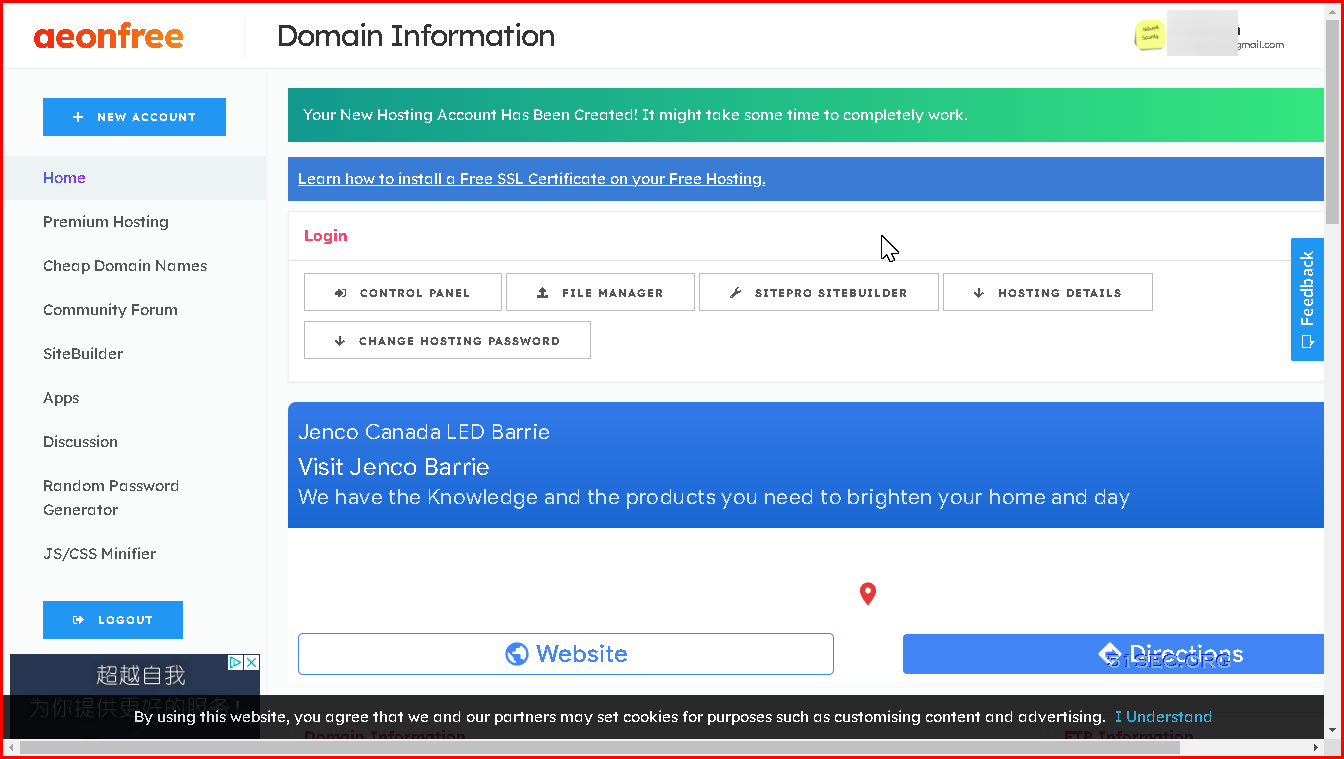Screenshot of the AonFree Website Displaying Domain Information

The image is a screenshot of the AonFree website, which provides domain information. The entire picture is bordered by a red line, highlighting the contents within. The website itself has a clean, white background.

At the top left, the logo "AonFree" is prominently displayed, featuring a color gradient transitioning from red to orange. To its right, the heading "Domain Information" is written in bold black text. In the upper right corner, some information is obscured by a light gray box.

Below the AonFree logo is a detailed navigation menu. The menu items are listed in blue text with various options:
1. New Account
2. Home
3. Premium Hosting
4. Cheap Domain Names
5. Community Forums
6. Site Builder
7. Apps
8. Discussion
9. Random Password Generator
10. JS/CSS
11. MiniFire

The menu also includes a blue "Logout" button. Beneath the menu is a navy advertisement with some white Chinese text that is truncated at the edge of the screenshot.

Centrally located on the page are links for user options including:
- Login Information
- Control Panel
- File Manager
- Site Pro Site Builder
- Hosting Details
- Change Hosting Password

Further down, the site shows website options or directions for "Genco Canada LEDBerry" with a promotional tagline: "Visit GencoBerry. We have the knowledge and the products you need to brighten your home and day."

Overall, the screenshot captures a comprehensive layout of the AonFree website, emphasizing domain information and multiple user navigation options.